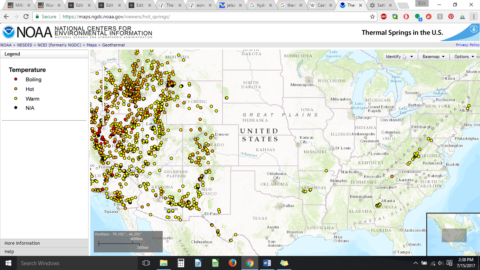The image features a detailed visual document from the National Centers for Environmental Information (NCEI). In the top left corner, the NCEI logo is displayed, with the recognizable NOAA icon—a light blue circle with a darker blue slice at the top. To the far right, the main header reads "Thermal Springs in the U.S." in black text against a white background.

Beneath the header, there's a narrow gray strip containing some hyperlinks labeled "NOAA," "NCEI" (possibly), and a note that the organization was formerly known as "NIGDC." Below this strip, additional links are listed: "next maps" and "geothermal."

On the left side of the image, a legend is presented in gray with black text. At the top, it states "Legend," followed by a section labeled "Temperature" in larger black font. Four colored dots are shown below:

1. Red dot with the label "Boiling."
2. Orange dot with the label "Hot."
3. Yellow dot with the label "Warm."
4. Black dot with the label "N/A" (indicating no thermal activity).

To the right of the legend, a map of the United States highlights the distribution of thermal springs. The map shows that most thermal springs are concentrated on the west coast, particularly in Nevada, Utah, California, and Arizona. There are a few exceptions with two yellow dots in eastern New York, several yellow dots along the right side of West Virginia, three yellow dots in Arkansas, and three yellow dots on the far left side of Georgia. Overall, the map provides a comprehensive visualization of thermal spring activity across the country.